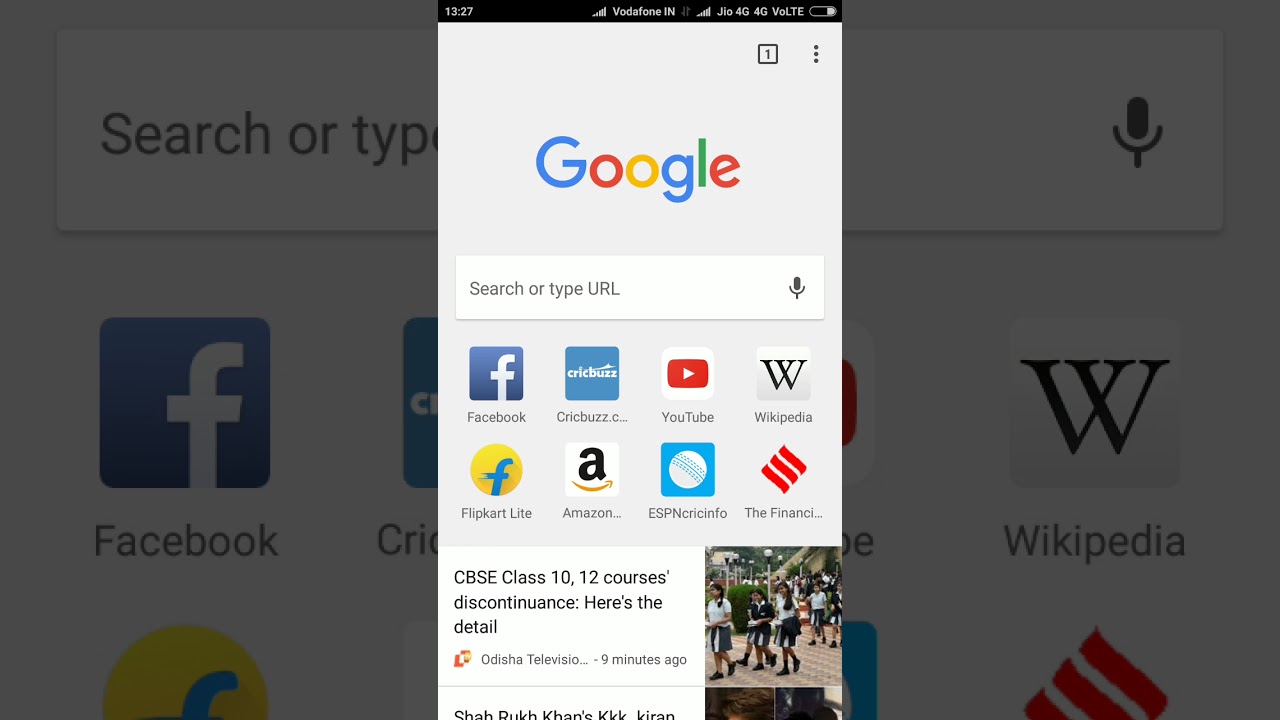The image depicts a smartphone screen as its primary focus. At the very top left corner, the time is displayed as 13:27. Next to it, the network signals for Vodafone IN and JIO are visible, both showing 4G connectivity and the presence of VoLTE (Voice over LTE). Central to the screen is the colorful Google logo, featuring the letters "G-O-O-G-L-E" in a mix of blue, red, yellow, and green.

Directly below the Google logo is a prominent search bar with a microphone icon to its right, and the text "Search or type URL" inside. Beside the search bar, a small square with the number "1" and three vertical dots is located in the upper right hand corner.

Scrolling down, one can notice various symbols and app icons. The Facebook symbol is easily recognizable with a capital "F." The Wikipedia icon features its traditional "W" above the word "Wikipedia." Other visible icons include YouTube, Flipkart Lite, Amazon, ESPN, Sorenfo, and The Financial.

Additionally, the screen shows a news-like notification about "CBSE class 10, 12 courses discontinuous" with further details available. This notification appears to have been posted 9 minutes ago. Below this, there's an image of what seems to be schoolgirls in uniform exiting a school building, hinting at a news story related to education.

The overall background is predominantly white, which makes the colorful elements and numerous icons stand out vividly on the screen.